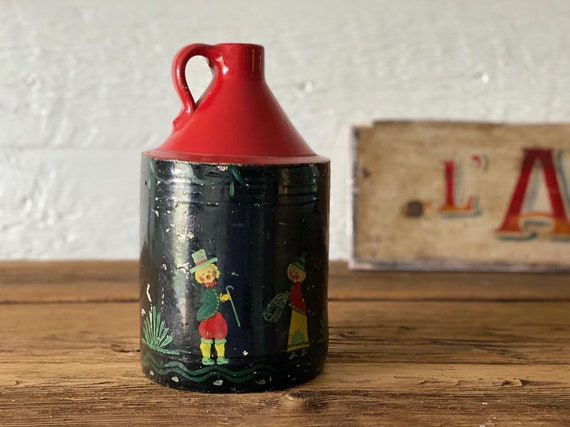Centered in the image is an ornate, black ceramic vessel with a red top and a red handle, placed slightly off-center on a brown, wooden surface, possibly a table or floor. The vessel features intricate artwork depicting two individuals adorned in yellow pants, red shirts, green robes, and green shoes. Both figures have yellow hair and wear distinct green hats. There are additional green spots and a green plant design on the vessel. The background is a white wall, providing a clean, neutral backdrop. To the right of the vessel, there is a partially visible wooden sign with the text "L'A" in red letters. The setting has an old-fashioned, rustic feel, reminiscent of a farmhouse. The high-quality image highlights the vivid colors of red, black, yellow, green, brown, and white.